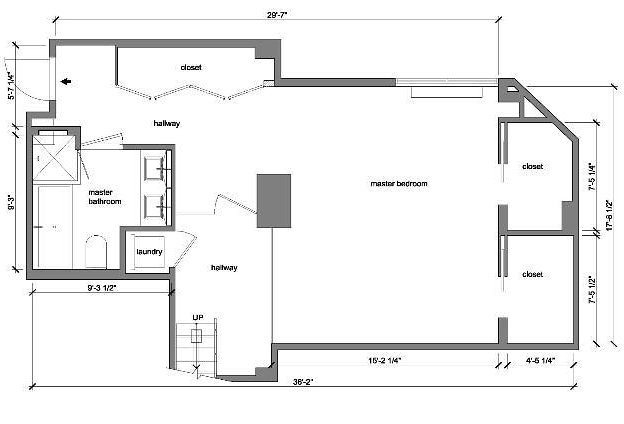This detailed photograph showcases a meticulously drawn blueprint of a single-story house. The house extends 36 feet 2 inches at its longest dimension and 29 feet 7 inches along the other, wider side. The structure features a cutback at the front, measuring 17 feet 8.5 inches. The rear of the house reveals two distinct sections, with one part measuring 9 feet 3 inches and the other 5 feet 7.25 inches.

The blueprint details a master bedroom, which includes not one, but two closets, and an adjacent master bathroom equipped with dual sinks, a bathtub, and a toilet. In addition, the layout incorporates a hallway leading to a staircase and another hallway accessing an extra closet and a laundry area.

A notable feature is an unaccounted-for space near the master bedroom, initially mistaken for a shower area. This space likely houses utility components, such as a water tank, providing a functional behind-the-scenes element to the house design.